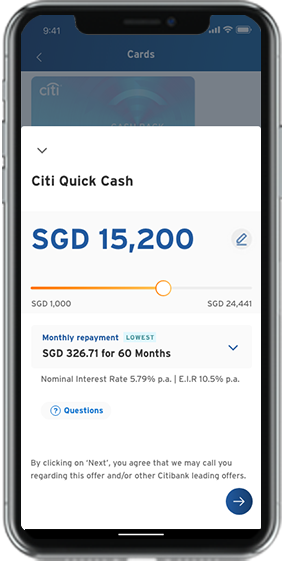The image depicts a smartphone screen with a gray-to-black gradient outer outline. A large pop-up window dominates most of the screen, leaving the visible screen area that isn't covered by the pop-up in a dark green shade. The rectangular pop-up window has a light gray background. 

In the top left corner of the pop-up is the end of a black arrow pointing downward, and adjacent to it in black text is "CityQuickCash." Below this, in blue text, it shows "SGD15,200." There's a small gray circle featuring a blue pen icon to the right.

The pop-up also includes an orange bar indicating a progress measure, spanning horizontally across the window. On the left side in black text, "SGD1000" is noted, while further right, an amount of "SGD24,441" is displayed. Below the orange bar, in blue text, it states "Monthly Payment," followed by a light teal box containing the word "Lowest."

Continuing in black text, the pop-up details "SGD326.71 for 60 months," followed by "Nominal interest rate 5.79% P.A. / E.IR.10.5% P.A." Towards the bottom of the pop-up, a gray oval button labeled "Questions" is highlighted in blue text.

At the very bottom, in black text, there's a disclaimer: "By clicking on 'Next' you agree that we may call you regarding this order and/or other CitiBank lending offers."